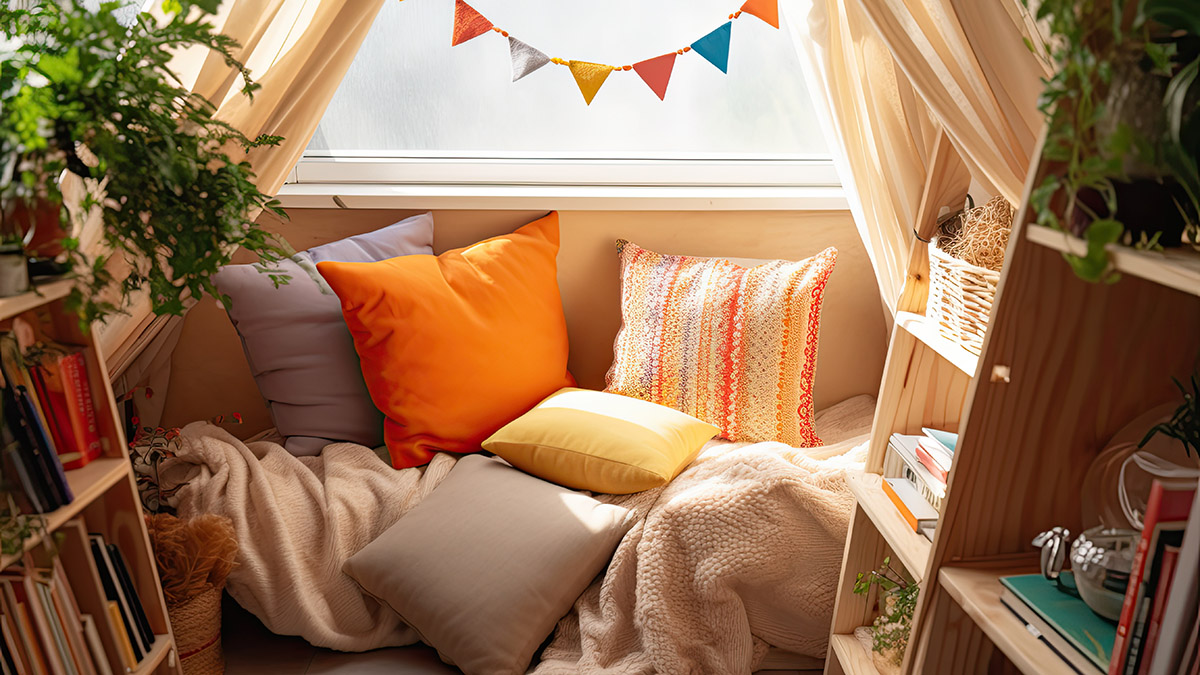In this cozy indoor scene, we see a small, sunlit reading nook centered around a white-framed window. A vibrant multi-colored pennant banner, featuring an array of colors such as red, orange, yellow, green, and white, hangs from the right side of the window, drooping gracefully to the left. Flanking the window are soft white curtains elegantly swooping outwards.

Below the window, a comfortable bench is adorned with a soft white blanket and a collection of five square pillows, each with distinct colors and patterns—gray, orange, yellow, purple, and a striped one in shades of gray, orange, and yellow. The bench is nestled between two wooden bookshelves made of unpainted wood. 

The left shelf houses an assortment of books standing upright and stacked horizontally, along with a green plant on the top. The right shelf mirrors this setup with similar books and another green plant, accompanied by a basket and various trinkets that assist in organizing the books. This serene corner, with its light brown and white tones, exudes a warm and inviting atmosphere perfect for relaxing with a good book.